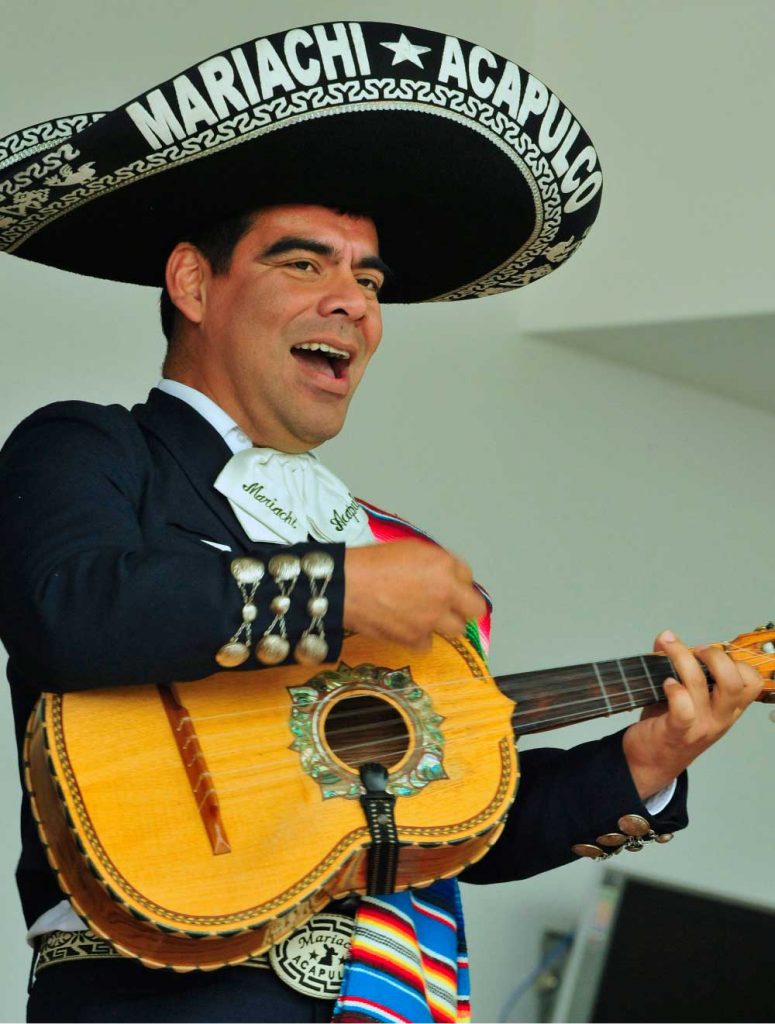The photograph captures a vibrant mariachi singer performing with passion. He wears a traditional black sombrero adorned with white detailing and the inscription "Mariachi Acapulco," accented by a prominent white star. The mariachi musician, with a strong face and dark, thick eyebrows free of any substantial beard, displays an expressive singing mouth, captured mid-performance. His outfit is meticulously traditional, featuring a white collared shirt beneath a black suit jacket studded with intricate silver buttons on the sleeves and ornate circular cufflinks. A white scarf knotted around his neck also displays the word "Mariachi".

He skillfully strums a small, possibly mandolin-like guitar that is embellished with a metallic floral pattern around the soundhole, his fingers poised on the fretboard to form notes. Draped over his shoulder is a colorful sash that adds a splash of vibrancy to his formal attire. A black and white belt that mirrors the design of his hat, bearing the phrase "Mariachi Acapulco," cinches his ensemble. The background is a plain white wall with a doorway discernible in the bottom right corner, subtly leading out of the scene. The image poignantly captures both the cultural richness and emotional intensity of the mariachi performance.